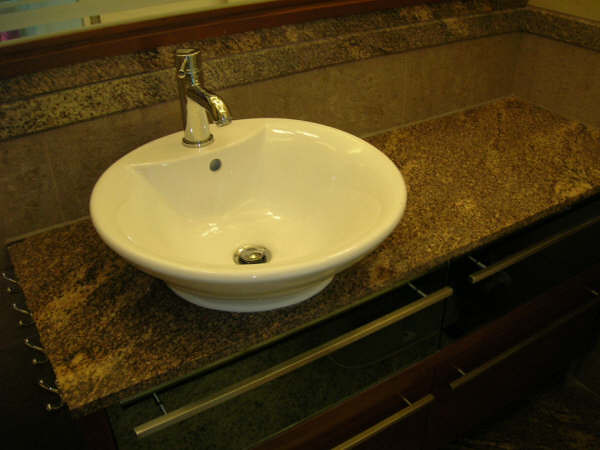This image features a modern bathroom vanity with a striking white, vessel-style sink prominently placed on top. The sink has a rounded design with an exposed base that tapers elegantly to a point. A sleek, stainless steel faucet complements the contemporary aesthetic. The vanity's surface is a luxurious, dark marbled material, approximately two inches thick, adding an element of sophistication. Below the sink, the vanity includes two spacious, black drawers, each adorned with long, two-foot horizontal bars that serve as stylish handles.